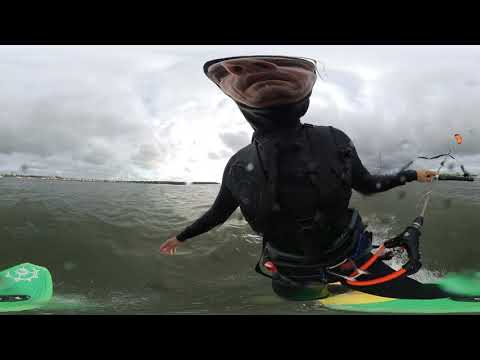In this outdoor image, a man is captured in a close-up, highly distorted by a fisheye lens, giving his face an exaggerated, vase-like shape with disproportionately large eyes, nostrils, and mouth. He has fair skin, possibly sporting a small beard or mustache, and wears an all-black wetsuit. Around his waist, there's an orange-colored string connected to a large clip, and a red item is seen in a pouch. His right arm is stretched out to the side, pointing towards the bottom left, while his left hand, holding onto a handle, is raised as if attached to a parachute-like apparatus in the background. He stands on a green surfboard with a yellow top half, on a body of water that appears to be a dirty, brownish-green or greenish-gray color. Dark clouds dominate the fairly cloudy sky, contributing to the overall moody atmosphere. The horizon shows some white and blue sky amidst the clouds, adding to the surreal and dynamic feel of the scene.